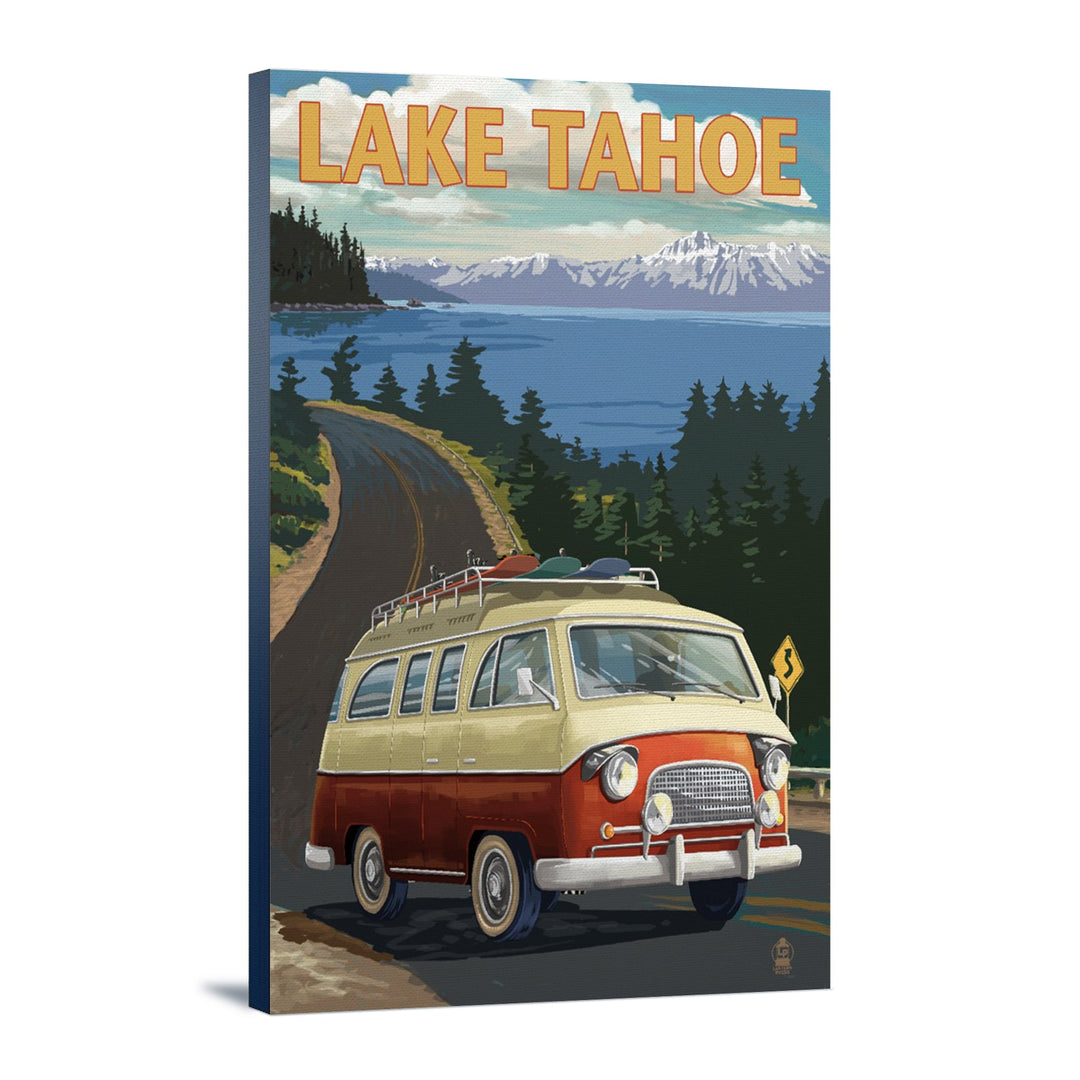This image appears to be a meticulously crafted vintage travel poster from the 1950s, promoting Lake Tahoe. At the top, the name "Lake Tahoe" is prominently displayed in bold, yellow uppercase text. The artwork presents a hand-drawn, retro National Parks style illustration, featuring a classic camper van with a red bottom and an off-white top, driving towards the viewer but slightly to the right. The van has equipment, likely snowboards or surfboards, strapped to its roof rack. The scene depicts the van on a road that winds around Lake Tahoe, set against a backdrop of snow-capped mountains and pine trees. The overall setting suggests a sunny day, capturing the picturesque beauty of Lake Tahoe with its serene lake, majestic mountains, and lush trees. The poster gives a nostalgic feel, with its 3D canvas-like display tilted slightly to the right, evoking a sense of adventure and exploration.